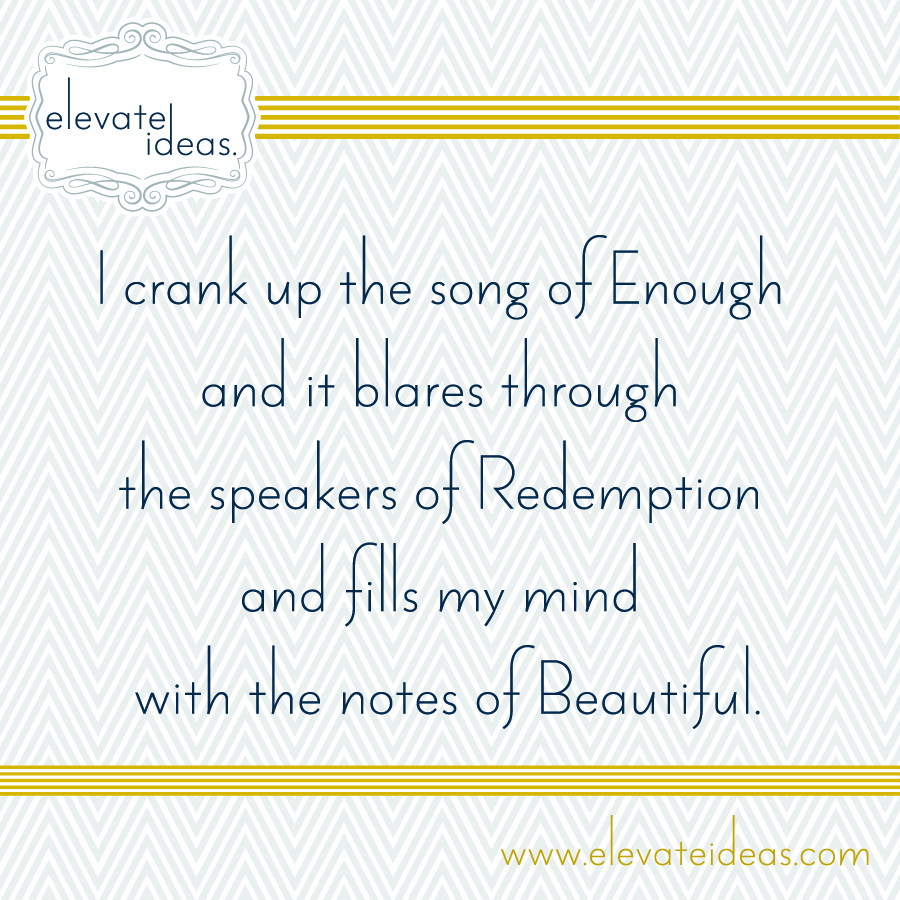This image features a sign with a detailed and vibrant design. The background showcases a pattern of diagonal gray and white lines interspersed with horizontal gold lines at the top and bottom. In the upper left-hand corner, there is a delicate design housing the text "Elevate Ideas" written in thin black letters. The central part of the image prominently displays a motivational quote in a mix of print and cursive-shaped black letters: "I crank up the song of enough, and it blares through the speakers of redemption and fills my mind with the notes of beautiful." Finally, in the lower right-hand corner, the text "www.elevateideas.com" is printed in gold, adding to the elegant aesthetic of the image.